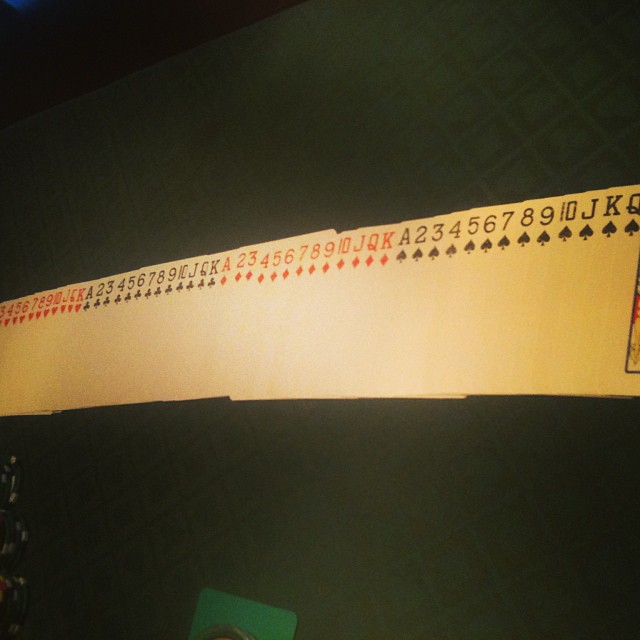A neatly fanned-out deck of playing cards is displayed on what appears to be a green felt card table. The cards are arranged face-up in a meticulously organized sequence from ace through king, grouped by suit and spread from left to right. On the far left, the hearts are shown, starting with the ace and followed sequentially up to the king, although only the first three cards are fully visible. Continuing to the right, the clubs are laid out in a similar fashion, followed by the diamonds. The sequence appears perfect until reaching the spades on the far right. Upon closer inspection, there is a noticeable anomaly: the spades deviate from the expected order, with the king appearing before the queen, after the jack and 10. This minor discrepancy stands out against the otherwise precise arrangement of the cards, adding an element of intrigue to the scene.